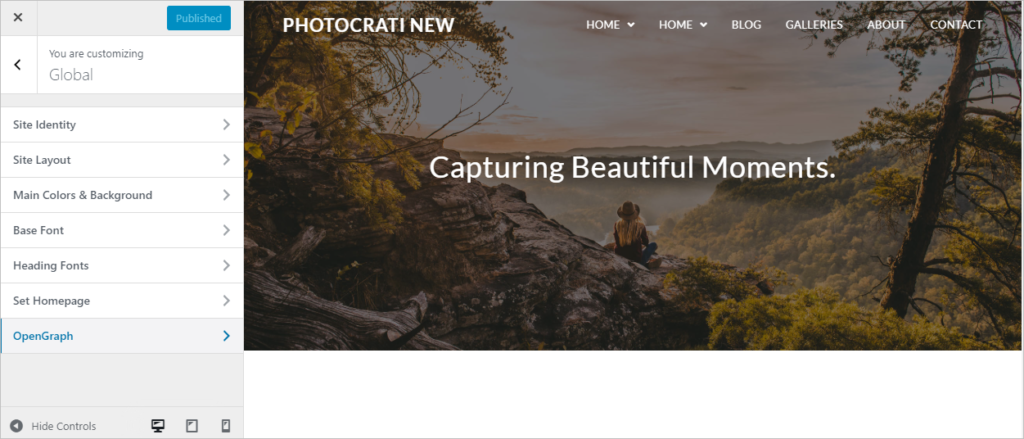This image showcases the user interface of a digital platform called "Photo Kratty New," although it's unclear if it's a website or a software program. The screen is divided into two distinct sections. The left-hand side features a gray box with an 'X' at the top, alongside a blue square that reads "Published." Below this, there's a list of customizable options, starting with "Site Identity," and continuing with "Site Layout," "Main Colors and Backgrounds," "Base Font," "Headings Font," "Set Homepage,” and finally, "Open Graph," which is currently highlighted in blue, suggesting it is the selected option.

The main section on the right displays a large, captivating image of a woman seated on a mountainside. She is looking out over a lush, forested landscape with trees in various shades of gold and green, viewed from behind. Bold white text across the image reads: "Capturing Beautiful Moments."

At the top of the screen, there is a navigation bar featuring categories such as "Home," "Blog," "Galleries," "About," and "Contact," with dropdown arrows next to "Home" and "Blog" indicating additional submenus. The bottom of the screen reveals a blank white space, spanning the width of the photo, suggesting an area for additional content or footer information.